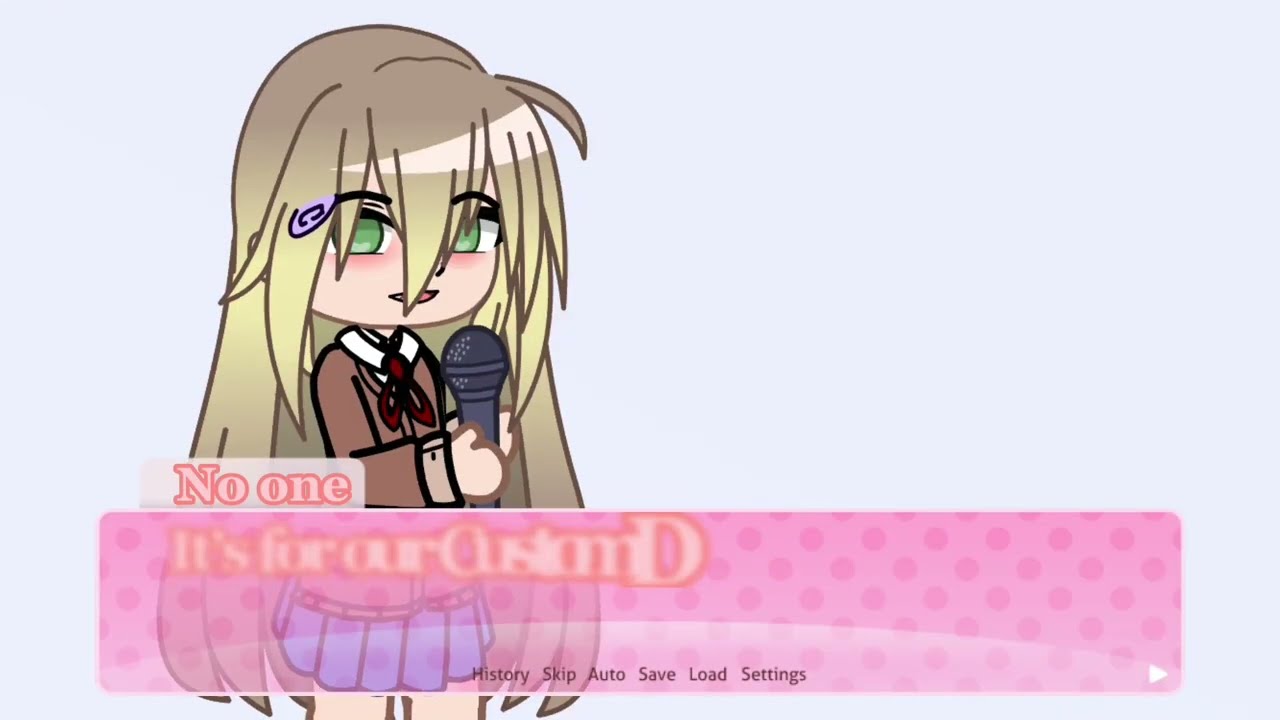The image features an anime-style cartoon character of a girl with distinct green eyes and extremely long, intricate blonde hair that falls down to her knees, styled with spikes and angles, and a purple hair clip. She has a round face partially covered by her hair, and she is holding a black microphone in her hands. She is dressed in a brown school uniform. The background of the image is a light blue or lilac color.

This girl is positioned towards the left side of the image. Below her, a pink rectangular bar with darker pink polka dots runs horizontally across the bottom. This bar has somewhat translucent properties, making part of the text behind it difficult to read. The visible portion of the text on the bar reads "No one is for R," with additional text obscured. Below this bar, clear text reads "history," "skip," "auto," "save," "load," and "settings." On the right-hand side of the bar, there's a white play arrow. This suggests that the image is likely a screenshot from a visual novel game or an interactive web page.